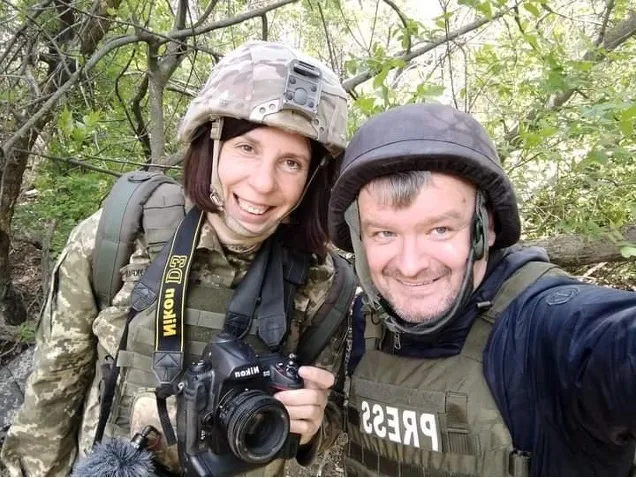In this image, a man and a woman are taking a selfie together in what appears to be a woodsy, forested area. The woman is on the left and is a white female with short, medium-length brown hair. She is wearing military-style gear that includes a hard hat made of fatigue fabric, army fatigues, a bulletproof vest, and a backpack. Draped around her neck is a large black Nikon camera, identifiable by the camera strap. The man on the right is also a white male, sporting a black hard hat and a black hoodie underneath a similar bulletproof vest. Notably, his vest has the word "PRESS" emblazoned in white, identifying him as a media professional. He has grayish hair and a happy smile as he holds the camera to take their photo. Both appear to be news reporters, likely in a war zone or conflict area, based on their attire and surroundings. The backdrop is rich with green leaves and branches, enhancing the sense of their wild or jungle setting.